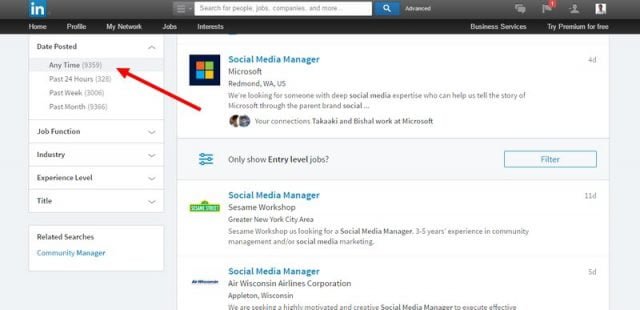Here is a cleaned-up, detailed descriptive caption for the given image:

---

The image is a detailed screenshot of a LinkedIn job postings page, showcasing several available positions. At the very top, a gray border frames the header of the page. The upper left corner features the LinkedIn logo - a blue square containing the white 'IN' letters.

Moving rightward from the logo, there is a prominent search bar labeled "Search for people, jobs, companies and more" accompanied by a clickable blue search icon. An adjacent white text "Advanced" offers further search options. On the right side of the header, there are icons for notifications, messages, and the user profile.

Below the header, a black bar provides navigation options: Home, Profile, My Network, Jobs, and Interests on the left, with Business Services and "Try Premium for Free" on the far right.

The left section of the page includes a white dropdown box for filters, displaying options such as "Date Posted" with selections for Any Time, Past 24 Hours, Past Week, and Past Month. Additional filters for job function, industry, experience level, and title are also visible. A red arrow has been photoshopped in, pointing to the 'Any Time' option. Below the filters, there is a "Related Searches" box displaying "Community Manager".

On the right-hand side, three job postings for the position of Social Media Manager are listed. The first position is at Microsoft located in Redmond, WA, indicated by the Windows logo. The second position is at Sesame Workshop in the New York City area, denoted by the Sesame Street logo. The third listing is for Air Wisconsin's Airline Corporation in Appleton, Wisconsin.